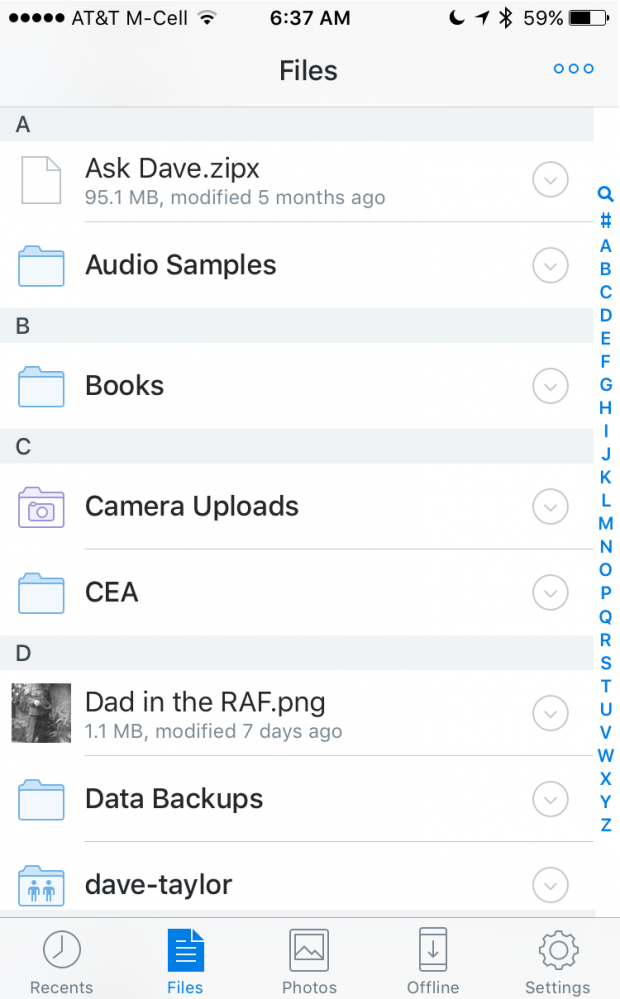The image displays a phone screen with the "Files" app open, featuring various folders and files. At the top left, five black circles indicate the signal strength, labeled "AT&T M-Cell" next to a signal icon. The time is shown as "6:37 AM." On the top right, a partial moon icon is accompanied by an upward arrow, indicating a 59% battery level. 

Below the time, the word "Files" appears on the left, aligned with three blue-outlined circles on the right. 

The list begins with:
1. **A** - "AskDave.zipX" featuring a gray, folded-paper icon, sized at 95.1 MB, last modified five months ago. A download arrow and a blue search icon are present.
2. **Audio Samples** - Represented by a blue folder icon.
3. **B** - "Books" with a similar blue folder icon.
4. **C** - "Camera Uploads" with a purple camera icon.
5. **CEA** - Indicated by the recurring blue folder icon.
6. **D** - "Dad in the RAF.png," a 1.1 MB file modified seven days ago, displayed alongside a black-and-white photo icon.
7. **Data Backups** - Another blue folder icon.
8. **Dave-Taylor** - A blue folder icon with two overlapping people icons.

At the bottom, navigation options include "Recents," "Files," "Photos," "Offline," and "Settings." "Files" is highlighted in blue with a blue square icon with folded white lines. "Recents" shows a gray clock outline, "Photos" displays a photo icon, "Offline" presents a phone with a downward arrow, and "Settings" involves the typical settings icon.

The right side of the screen lists alphabet letters A through Z in blue, starting from "Audio Samples."